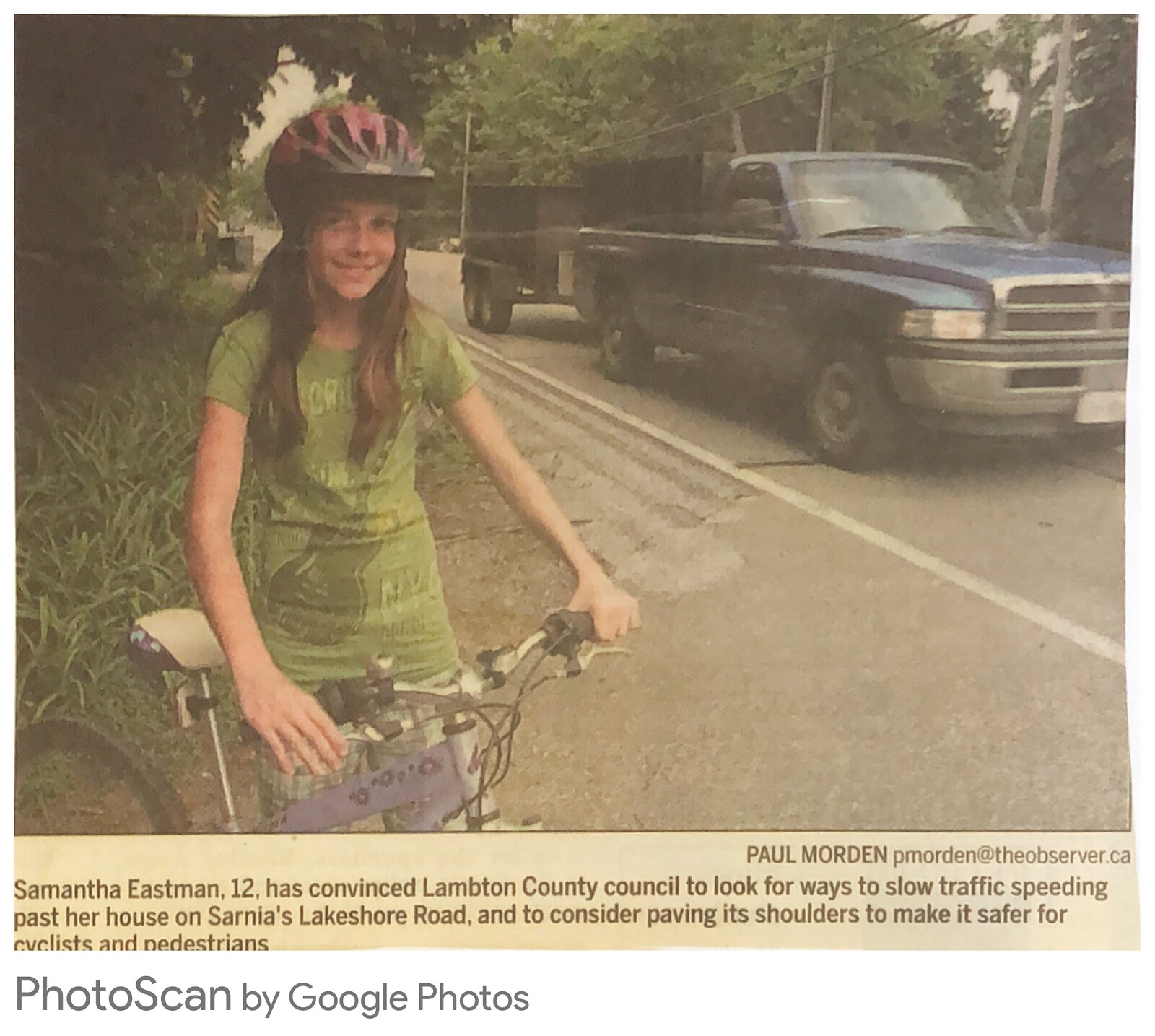The image is a color photograph from a slightly aged newspaper, possibly from the 1970s or early 1980s, as the colors appear a bit faded with a yellowish hue. The main subject of the photograph is a young girl named Samantha Eastman, 12 years old, standing beside her bicycle on the bottom left of the picture. Samantha is wearing a green T-shirt, purplish pants, and a black helmet with pink stripes on the back, her silver-brown hair flowing to her shoulders. She is positioned next to her bicycle, which features black handlebars and a white seat. In the background, there is a blue pickup truck towing a trailer along a road, and the scene is framed by trees and grass on one side. The caption details that Samantha has successfully convinced Lambton County Council to address the issue of speeding traffic near her house on Sarnia's Lakeshore Road and to consider paving the shoulders to improve safety for cyclists and pedestrians. The photograph is credited to Paul Morden of The Observer, with additional annotation indicating it was scanned using Google Photos.